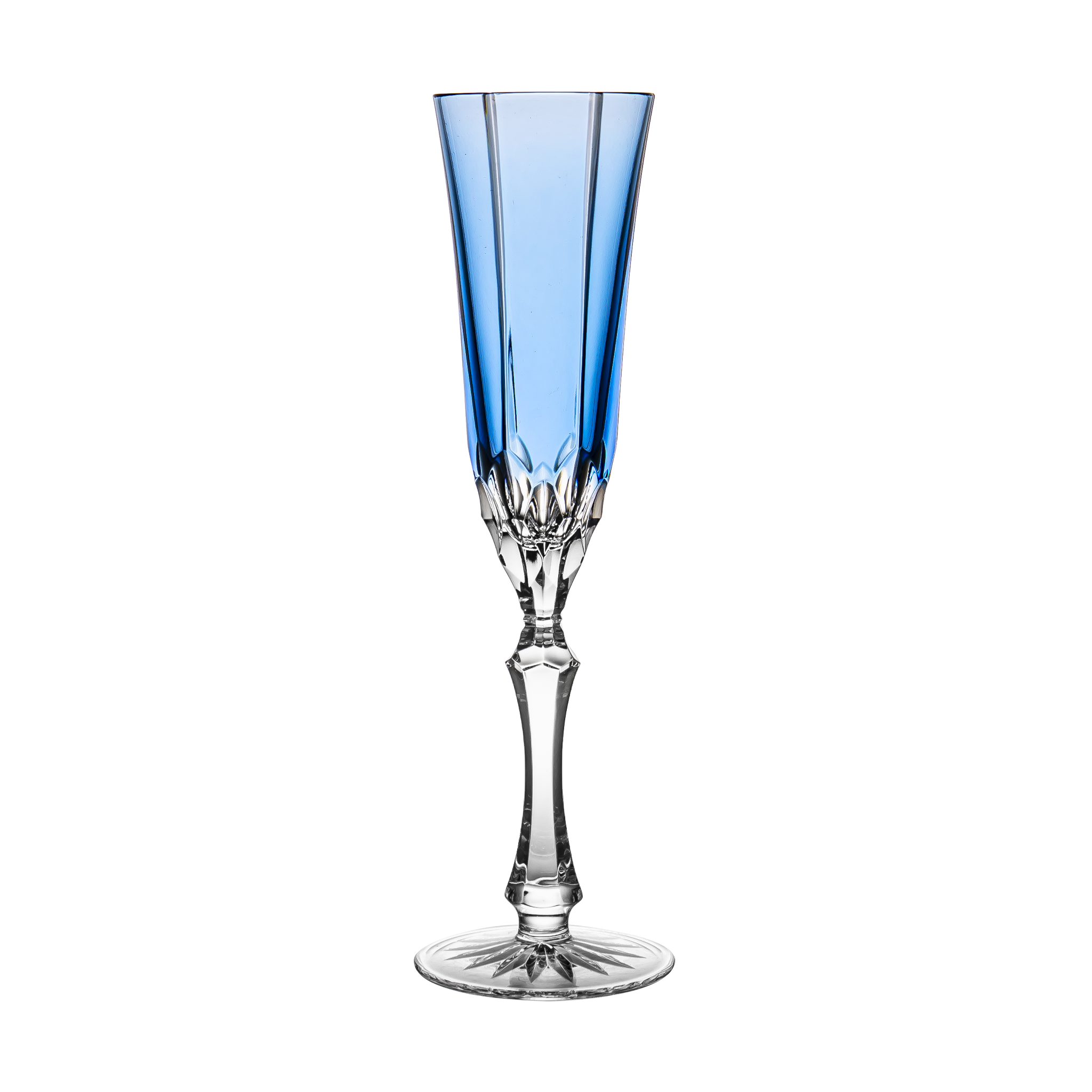This image showcases a stunning, intricate champagne glass set against a pristine white background that accentuates its clarity. The glass is crafted from crystal and features a royal blue to light blue gradation from the top down to the chalice-shaped holder. The top part of the glass, which flares out like a flute, is not perfectly round but appears to have an octagonal shape, giving it distinct flat edges. The holder smoothly transitions into a slender, clear crystal stem and a medium-sized, circular base. The base is etched with a delicate floral or star pattern, resembling petals emerging from the stem. The entire piece has an angular yet elegantly curved design, highlighting the meticulous craftsmanship that makes this glass especially captivating and unique.